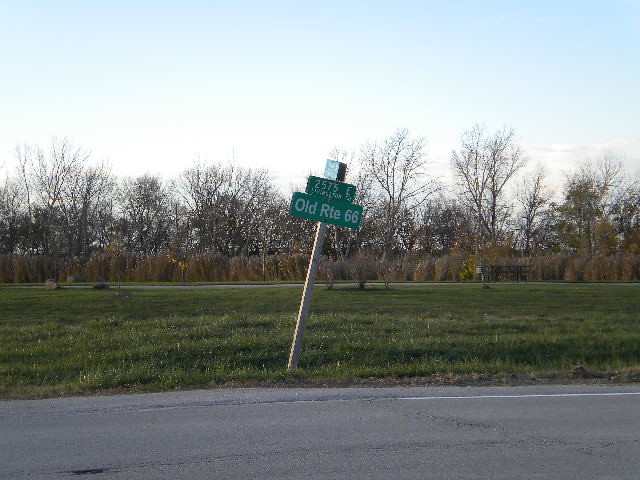The photograph, taken during the day, captures a street scene with a slightly cracked, gray pavement at the bottom. A white line runs along the edge of the road. Beyond the road is a large grassy field with varying heights of green grass, stretching halfway up the image. Slightly left of center stands a slightly bent wooden pole with a green street sign. The sign, attached to a white post, displays "2575 East" in a smaller white rectangle above a larger one that reads "Old RTE 66." In the background, there is a secondary concrete road, followed by a row of brownish-green bushes. Further back are tall trees, mostly bare with occasional leaves, silhouetted against a sky transitioning from white near the horizon to blue at the top.